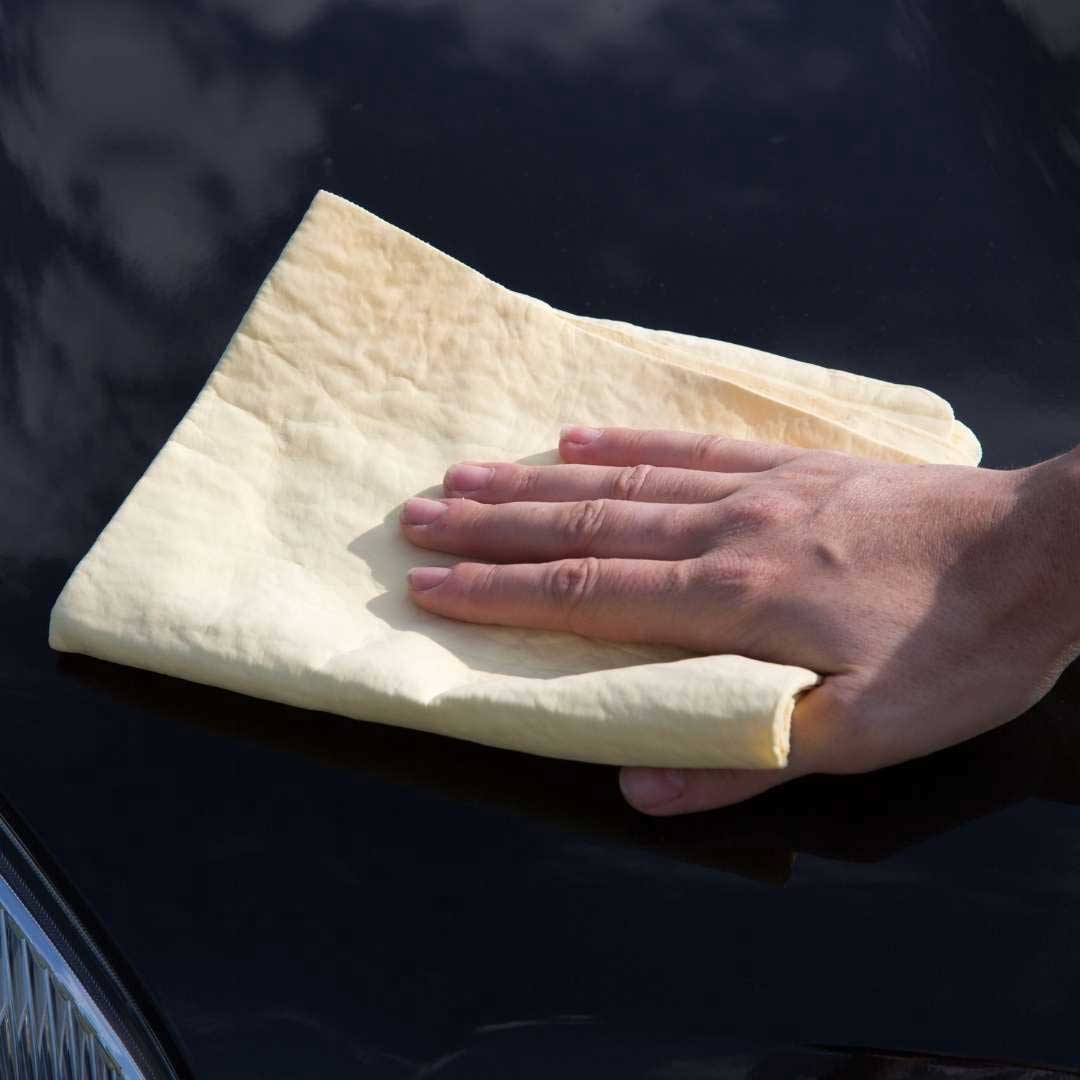In this brightly lit outdoor photograph, a male hand, light-skinned or white in complexion, extends from the right side of the image. The hand grips a neatly folded, light yellow or light tan chamois cloth, which appears brand new with no creases. The thumb is positioned underneath the cloth, suggesting movement as if wiping down or polishing the glossy black hood of a car. The hood reflects the sky above, adding a touch of visual depth to the scene. In the lower left corner, a small portion of the car's front grille is visible, emphasizing the focus on the cleaning action. The background remains nondescript, ensuring that the primary attention is on the hand and the chamois in the process of detailing the car.